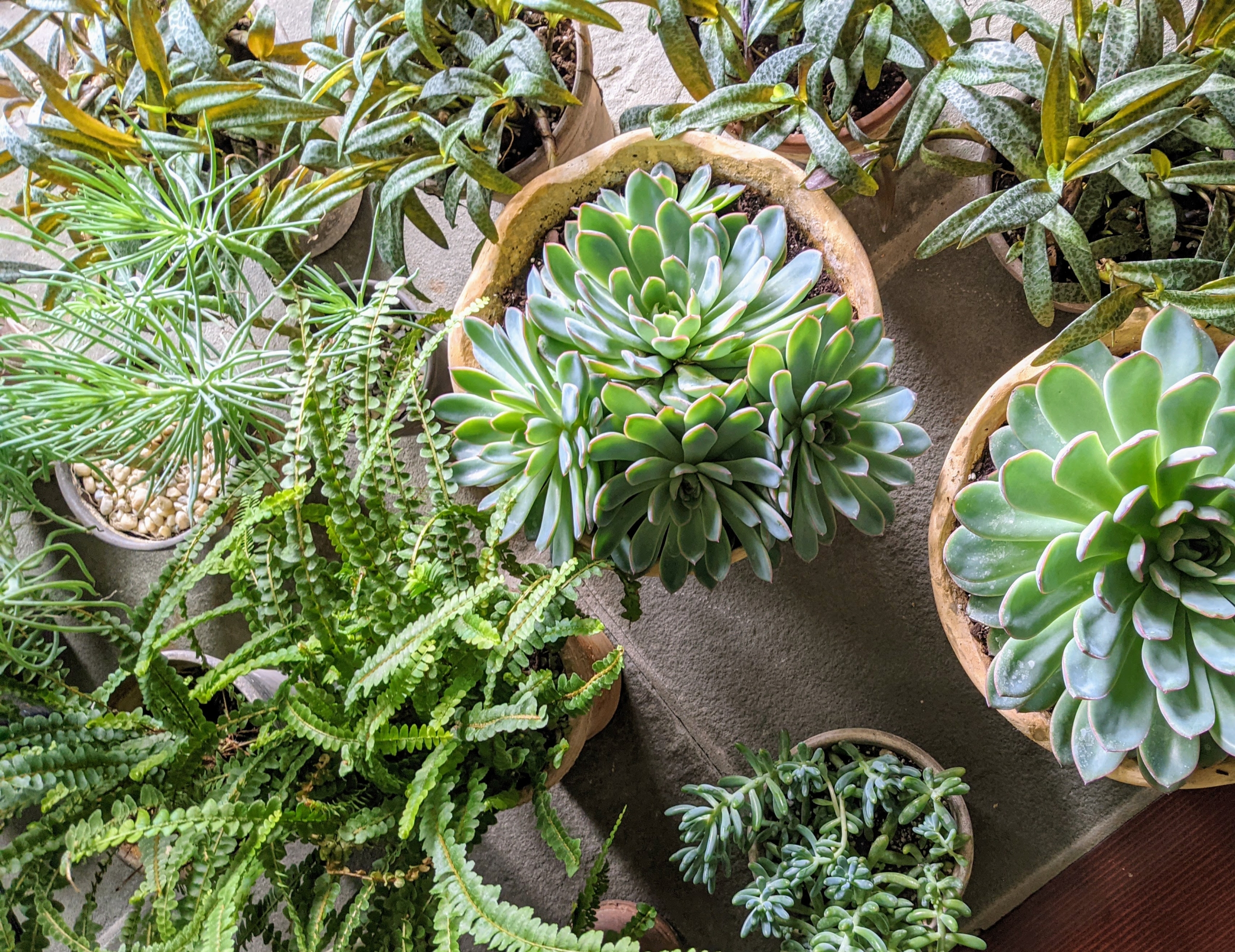This overhead photograph showcases an indoor display of various potted plants arranged on a wooden table with gray mats underneath. At the center of the image, there's a small green cactus resembling flower buds, with a similar cactus to its right. Surrounding these cacti are multiple potted succulents of different species, some growing low to their pots, while others extend upwards and outwards. The top section of the photo features dark brown pots containing plants with thin green leaves, mottled with white. To the left, green spider plants are visible, and in the bottom left corner, two pots house sprawling fern plants. Additionally, a single pot in the center towards the bottom holds a plant with branches reminiscent of a pine tree, but thicker and more rubbery. The overall arrangement of plants demonstrates a variety of textures and colors, creating a lush and diverse indoor garden scene.